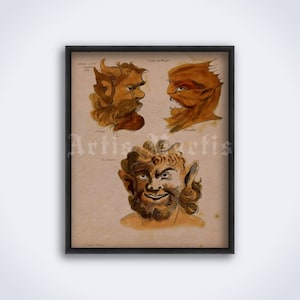The image shows a vintage-style artwork mounted in a black frame on a white wall, illuminated by light coming from the right side. The artwork is drawn on beige-colored paper, resembling parchment, and features three detailed illustrations of medieval, mythical beings with pointed ears and horns, suggestive of satyrs. The upper two sketches show side profiles—one facing left and the other facing right—while the bottom one displays a forward-looking figure with a beard and shaggy or curly hair, smirking with an evil grin. The artwork includes the word "Aeolus" and another word that appears to be "white." Additionally, there is a watermark across the drawing, which seems to read "Artist Martis." Despite its low resolution and slight blurriness, the piece stands out due to its unique and artistic depiction of these supernatural creatures.